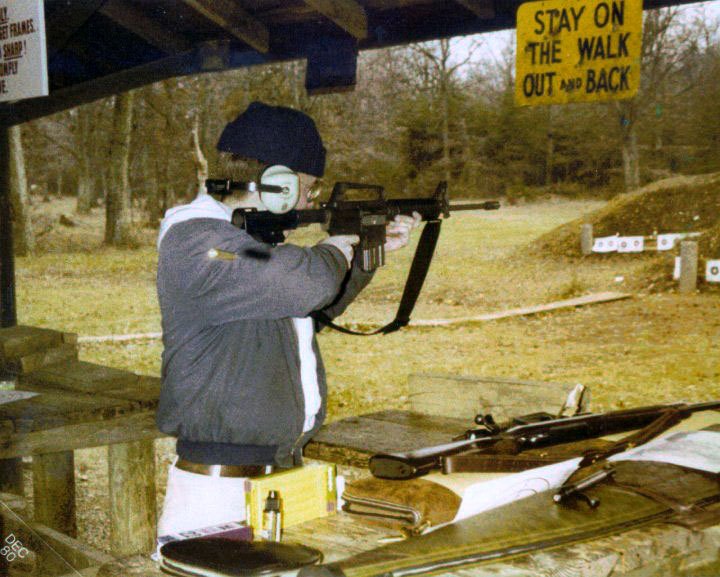The image depicts a grainy, likely Polaroid photograph taken at a shooting range in December 1980. In the center of the image, a focused man is aiming a black rifle. He is dressed in a gray jacket and light blue or white pants with a brown belt. He wears white earmuffs for protection. A blue cap or beanie covers his head. Situated in front of him is a wooden stand holding several other rifles. The background features a grassy area with a line of paper targets positioned on a small hill, and trees can be seen further back. Two signs are present: a white one in the top left corner and a prominent yellow sign at the top right corner with black text reading, "Stay on the walk out and back." An awning extends above the man, completing the scene.